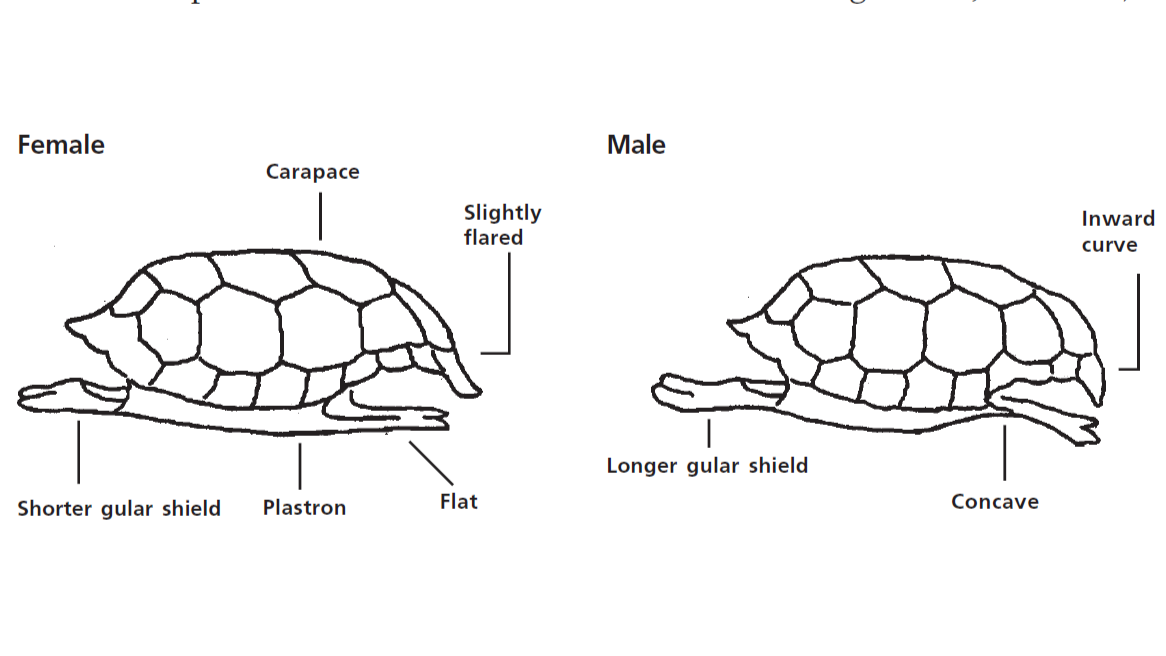The image consists of detailed black and white sketches comparing the anatomical differences between female and male tortoises. On the left side, labeled "female" in black text at the top, the sketch highlights several key features: the carapace, which is the top part of the shell, is identified and has a slightly flared edge on the right side. The gular shield, located at the front of the shell, is shorter and bends upwards before curving down. Beneath the shell, the plastron, or the bottom part of the shell, is labeled "flat." In contrast, the right side of the image is labeled "male." The male tortoise's shell, or carapace, has an inward curve on the right side. The gular shield in males is longer, and the plastron curves upwards, labeled as "concave." The sketches effectively illustrate these sexual dimorphisms, showcasing the distinct differences in shell structure and shape between female and male tortoises.